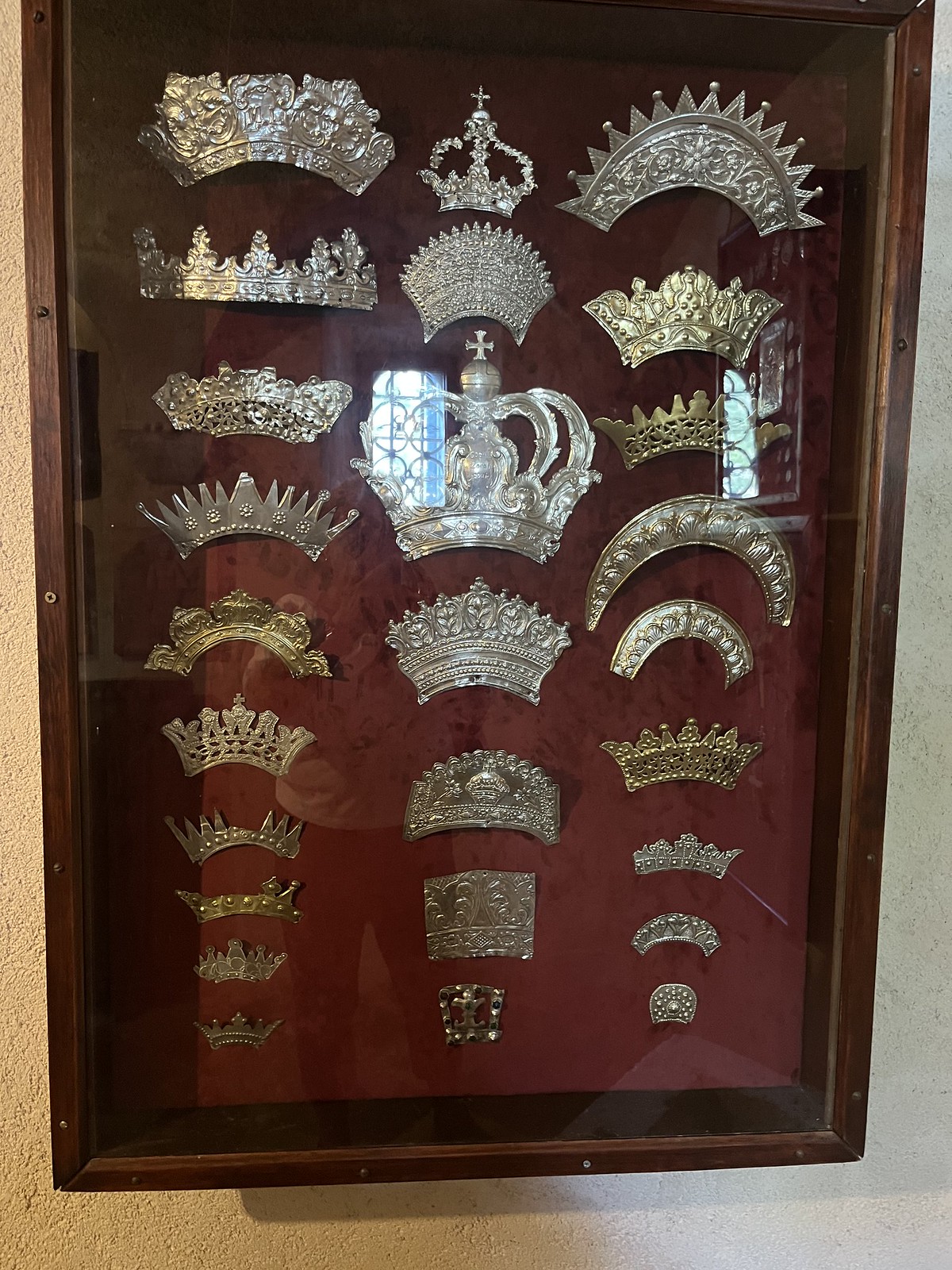This image shows a dark brown wooden display cabinet with a glass front, mounted on a textured cement wall that's light brown on the left and light gray on the right. Inside, the display case contains multiple ornately carved crowns and tiaras that descend in size from top to bottom. The crowns, mostly silver but with some darker and gold-plated variations, are arranged in three vertical rows against a dark red velvet backing. The left row contains ten crowns, the middle row has seven, and the right row has nine. The largest crown, in the center, features a cross and a circular base. The intricate designs include floral motifs, and as you move up the display, the crowns become larger and more elaborate. Reflections on the glass front show windows behind the photographer, adding a hint of blue or green to the scene. The image likely captures an exhibit in a historical museum showcasing royal artifacts.